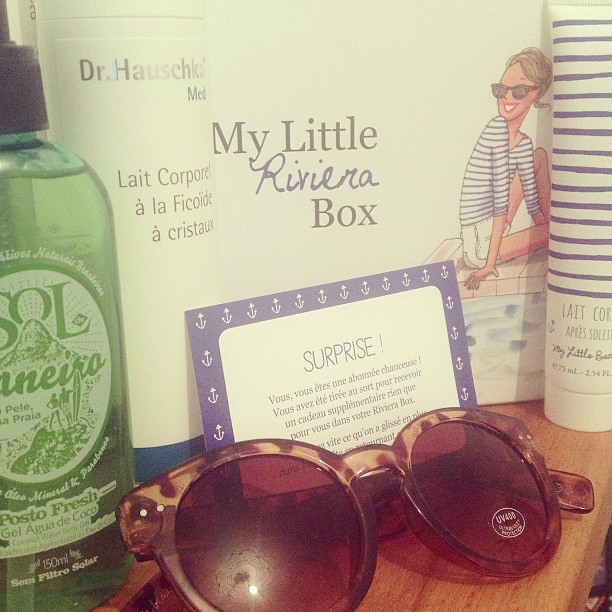This color photograph, though of average quality and resolution, captures a close-up of various beauty and lifestyle items displayed on a small wooden table. Dominating the foreground are a pair of plastic tortoiseshell sunglasses with round, light brown-tinted lenses. To the left of these sunglasses stands a tall, green bottle with white print, labeled "SOL" and featuring motifs of mountains and two people holding a surfboard. The bottle is described as containing a mineral-rich "Pasto Fresh Gel" infused with "Agua de Cocoa." Next to this green bottle, to the right, is a white bottle labeled "Dr. Hauschka Med," which appears to be a French product. 

In the background, there is an illustration on a packaging box that reads "My Little Riviera Box" in black text, with the word "Riviera" scripted in blue cursive. This box features a cartoon of a blonde woman lounging by a pool, wearing sunglasses and a striped shirt. Below this illustration lies a card with a white center framed by a blue border decorated with white anchors. The card prominently displays the word "Surprise" and contains additional text in French, which is partially legible.

This arrangement suggests an assortment of chic, possibly French, beauty and lifestyle products, all set against the rustic charm of a wooden tabletop.